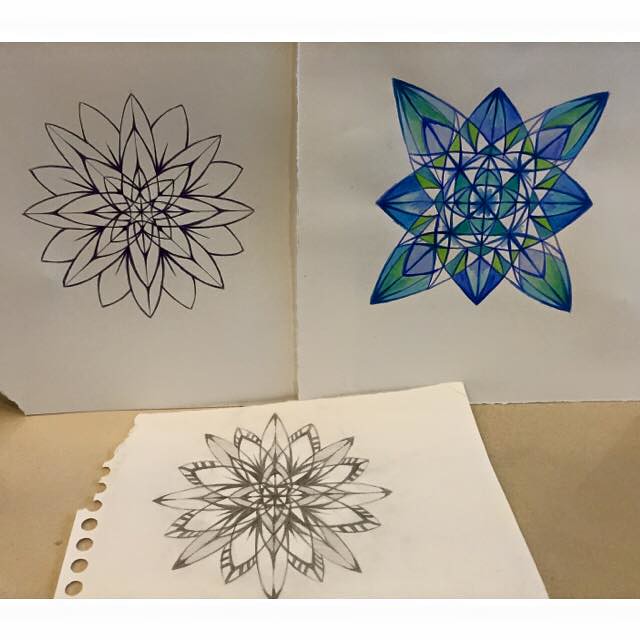This photograph showcases three intricate geometric drawings that resemble spirograph designs, all rendered on off-white paper. The composition features two drawings mounted on a wall and one positioned on the ground in the foreground. The wall-mounted drawings are placed symmetrically, with one on the left and one on the right. The drawing on the ground is centered between the two wall-mounted pieces. Notably, the paper of the foreground drawing has visible imperfections, including holes and a tear on its left side. The left-side wall-mounted drawing also exhibits damage, missing a portion from its bottom left corner. In contrast, the right-side wall-mounted drawing stands out with its vibrant blues and greens, depicting a complex configuration of a four-sided figure atop a four-petaled structure. The other two drawings are monochromatic, rendered solely in black and white.